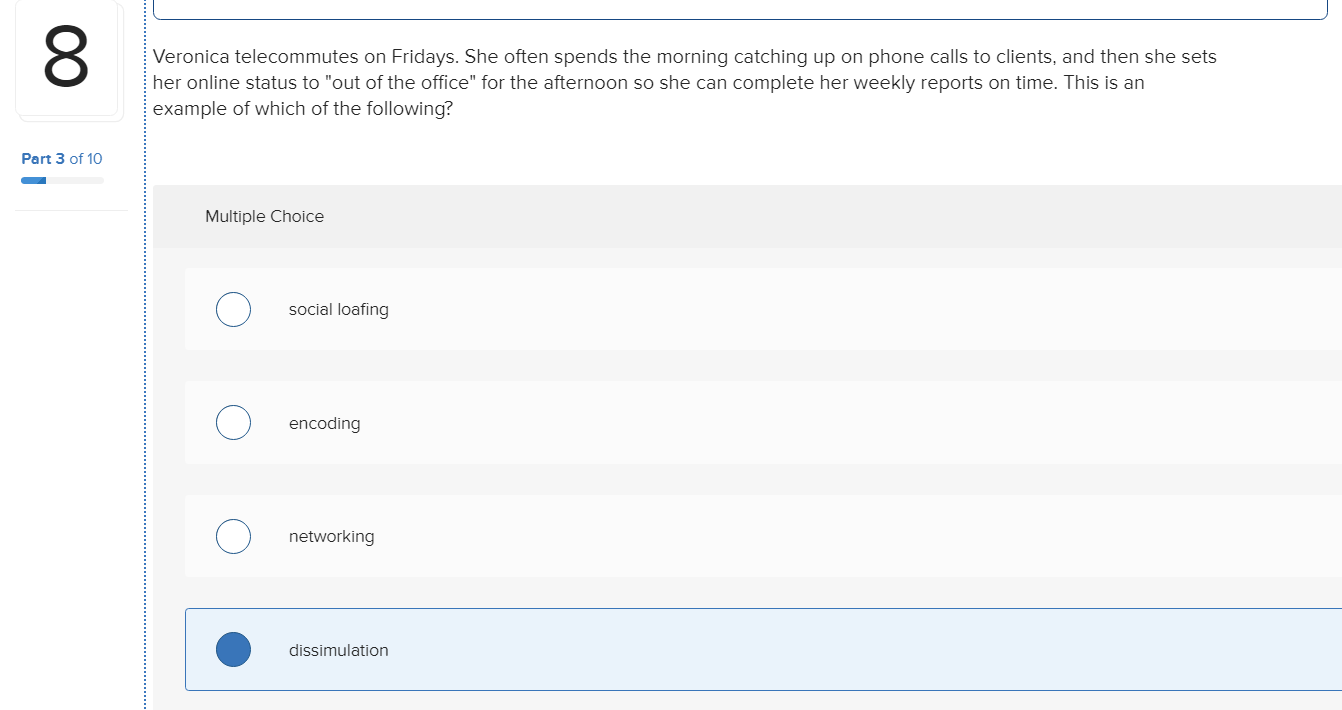**Screenshot Description: Multiple Choice Test Question Detail**

This image is a screenshot of a digital test interface, specifically showing question number 8, part 3 of 10. The screen features a clean, white background with distinct blocks dedicated to each question. Each question block consists of a white area where the question is presented and a blue area containing the answer choices.

For question 8, the prompt reads:
"Veronica telecommutes on Fridays. She often spends the morning catching up on phone calls to clients, and then she sets her online status to 'out of office' for the afternoon so she can complete her weekly reports on time. This is an example of which of the following?"

This question is followed by four multiple-choice options, each accompanied by a circular selection button. The options are listed in a darker blue color against the white background:
1. Social loafing
2. Encoding
3. Networking
4. Dissimulation

Notably, the circle next to "Dissimulation" is filled in with a cornflower blue color, indicating that this is the selected answer. Additionally, the area around the "Dissimulation" choice has a baby blue tint, further highlighting the selection against the otherwise white background.